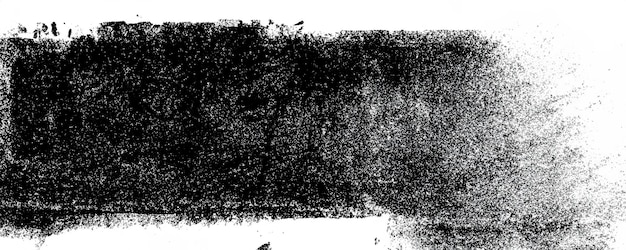This abstract image features a predominantly white background with an array of black dots and smudges arranged in a rectangular formation that extends from the left to the right side. The concentration of these black marks is heavier on the left side, gradually becoming lighter and more dispersed on the right, revealing more of the white background. In addition to the black dots, there are also faint white smudges intermingled. The pattern of the marks appears off-centered, creating an uneven yet intriguing visual effect. The overall impression is a dynamic contrast between light and dark, with no discernible text or clear depiction of objects, though it vaguely resembles a pipe and valve to some viewers.